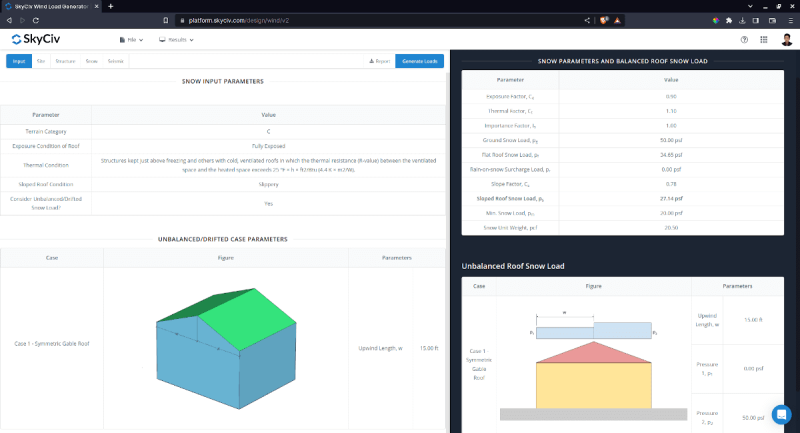The image showcases a webpage from a site named SkyCiv, as indicated by the logo positioned in the top left-hand corner. The browser appears to have a single tab open. Dominating the left side of the lower section, there is a three-dimensional, house-shaped object. This object features a green-colored roof, with blue sides and front. On the bottom right-hand corner, another house-shaped figure is visible, displaying a light red roof and yellow sides and front. The presence of these models suggests that the website pertains to building architecture or 3D modeling. Despite abundant information being present on the page, the text appears too small to read. Additionally, the top right-hand corner of the webpage displays a user's profile picture.